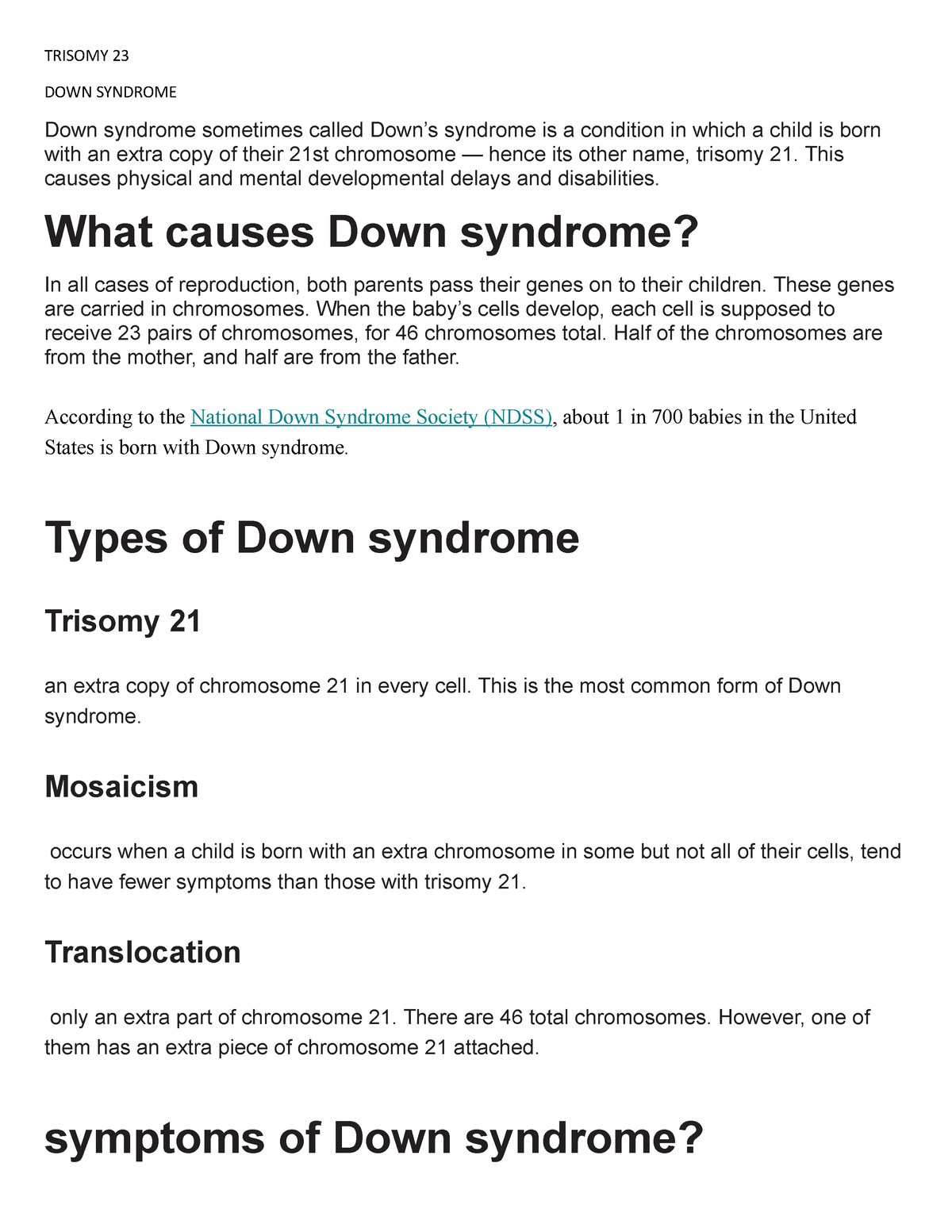This screenshot displays a detailed page about Down syndrome. In the upper left corner, there's small text reading "Trisomy 23, Down syndrome." Down syndrome, often referred to as Down's syndrome, is a condition where a child is born with an extra copy of their 21st chromosome, known as Trisomy 21. This results in physical and mental development delays and disabilities. In large black text, the question "What causes Down syndrome?" is posed. 

The text explains that during reproduction, both parents pass their genes to their child through chromosomes. Ideally, a baby's cells should receive 23 pairs of chromosomes, making a total of 46. Half of these chromosomes are inherited from the mother and the other half from the father. According to the National Down Syndrome Society (NDSS), which is highlighted in blue underlined text, 1 in 700 babies in the U.S. is born with Down syndrome.

The page proceeds to explain the "Types of Down syndrome" in large text:
- **Trisomy 21**: The most common form, where every cell has an extra copy of Chromosome 21.
- **Mosaicism**: Occurs when some cells have an extra chromosome, resulting in fewer symptoms compared to those with Trisomy 21.
- **Translocation**: In this case, there are still 46 chromosomes, but one has an extra piece of Chromosome 21 attached.

The section concludes with the heading "Symptoms of Down syndrome?" indicating further information on the symptoms is provided or implied elsewhere on the page.